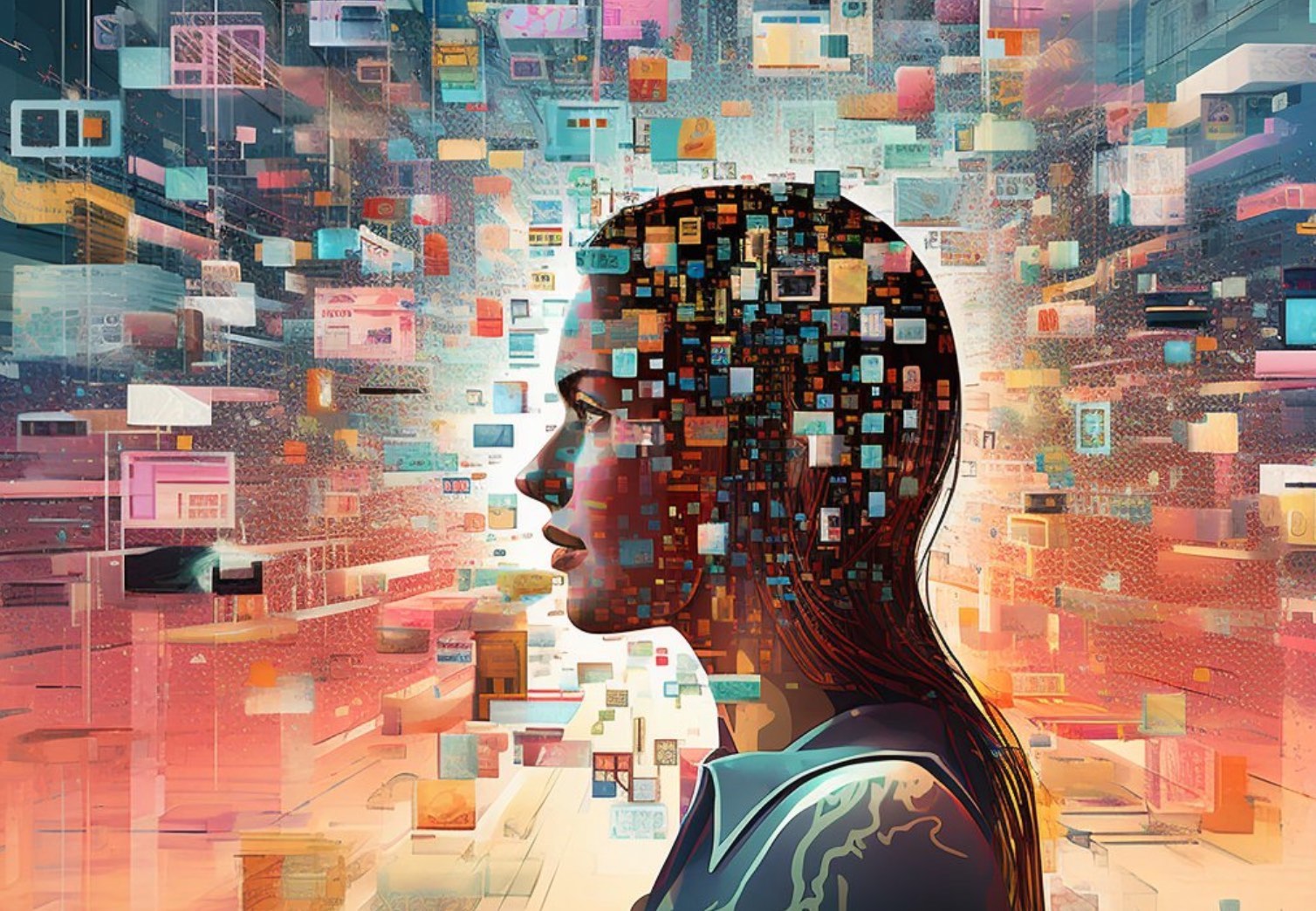The image is a vibrant, computer-designed artwork that evokes the feel of a conceptualized artificial intelligence or a vivid screensaver. At the center, a detailed portrait of a woman is depicted in profile, facing left. She has brownish-red hair cascading past her shoulders and wears a blue collared blouse. Surrounding her head, colorful squares and rectangles burst outward like an explosion of digital pixels, starting densely packed with vivid blues, purples, pinks, and yellows near her head and spreading out more sparsely as they reach the edges of the image. This emanation gives a sense of digital data dispersing into the surrounding space, with a white glow around her head transitioning into these vibrant hues, enhancing the surreal and dynamic nature of the artwork.